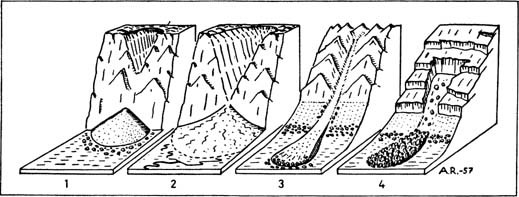The image appears to be an educational illustration from a book, depicting the process and stages of hilltop terracing through a series of four detailed, simple line drawings. Each drawing is labeled 1 through 4, and they sequentially show the transformation of a hillside. In the first drawing, the hillside is mostly intact but shows some sediment piling up at the bottom. The second drawing indicates a larger cut through the hillside with an increased silt deposit at its base. The third image further exaggerates this erosion, depicting a significant split down the middle of the hill with more sediment accumulation. Finally, the fourth illustration shows well-defined terrace steps cut into the hillside, with the most sediment collected at the bottom. The entire diagram is rendered in black and white with detailed stippling and line work used to convey texture and depth. Additionally, the letters "AR-57" appear on the right-hand side of the drawing, possibly denoting a reference or category.